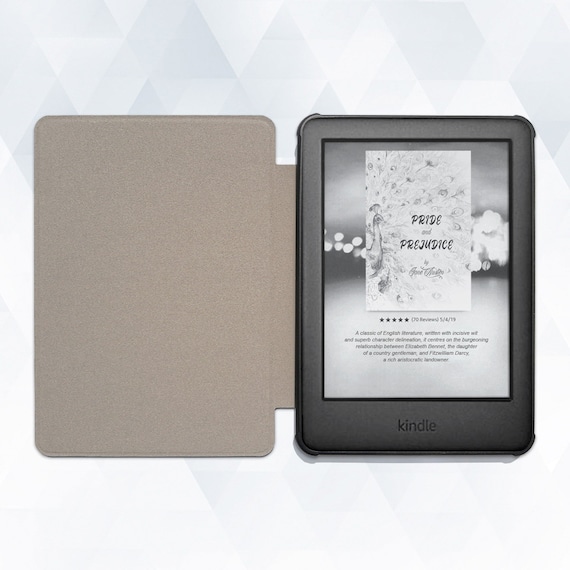The image is a detailed stock photo, likely intended for an online shopping website such as Amazon, depicting an old Kindle e-reading device encased in a protective cover. The Kindle, made of black plastic, features a matte black finish that appears soft in texture. It rests in a holder with a sandy brown flap that folds over the screen for added protection, reducing the risk of damage from drops or impact.

The screen of the Kindle displays the book “Pride and Prejudice,” showing its cover with an intricate peacock design, a brief description, and a five-star rating with associated black stars. The background of the Kindle's display utilizes a pattern of stars or flares to highlight the book's artwork. Below the screen, the brand name "Kindle" is clearly visible. Surrounding the Kindle, the overall background of the image is composed of gray and white diamond shapes, adding a professional, commercial feel suited for advertising purposes.